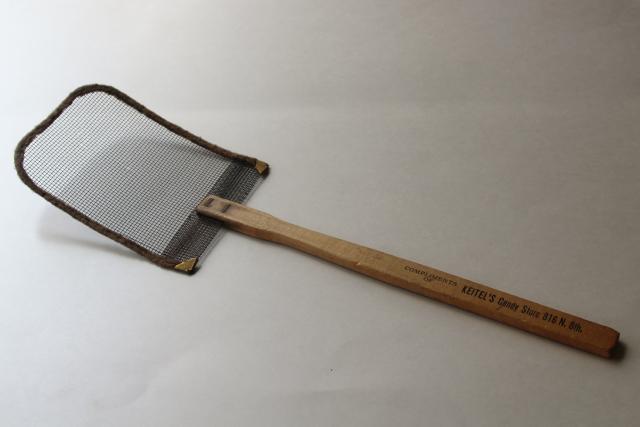The photo features a vintage fly swatter positioned on a plain white surface, with the business end oriented towards the upper left-hand corner of the image. The fly swatter comprises a long, flat wooden handle, secured with industrial staples to a nearly square mesh netting head. The mesh, made of black netting, is reinforced by a wire border and folded at the bottom for added rigidity. The netting has L-shaped brass brackets on the bottom corners for extra sturdiness. The handle bears stamped or stenciled lettering that reads, "Compliments of Keitel's Candy Store, 816 North 8th," suggesting it was likely a promotional item from the candy store. The image is slightly illuminated from the left, casting a gentle shadow to the right.